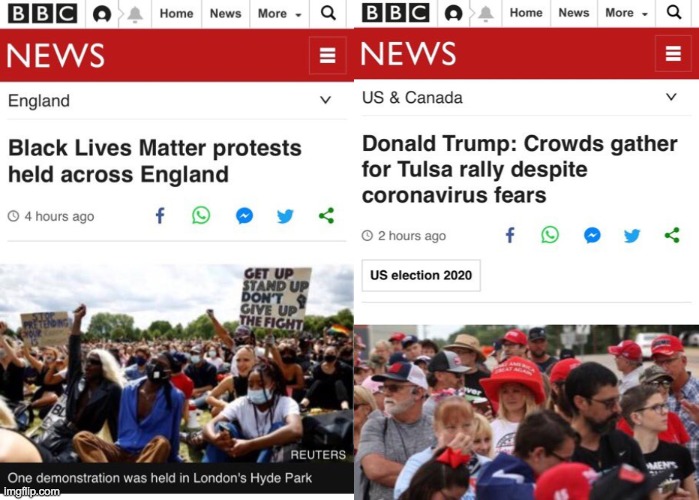This image is a detailed screenshot of two BBC News articles displayed side by side, either from a laptop screen or website view. At the top of both sections is the familiar BBC logo featuring black squares behind each white letter of "BBC." Below the logo, a prominent red banner with "NEWS" in bold, capitalized white letters spans across, with a vertical hamburger menu located on the top right corner of the banner. Underneath this banner, on the left-hand article, the headline reads "Black Lives Matter protests held across England," categorized under "England" with a drop-down menu on the right side. In contrast, the right-hand article is categorized under "US & Canada" and has the headline, "Donald Trump: Crowds gather for Tulsa rally despite coronavirus fears," also featuring a drop-down caret on the right side.

Each article indicates the time since it was posted: a greyed-out clock icon on the left shows the England article was posted four hours ago, whereas the US & Canada article was posted two hours ago. Below this, the US & Canada article displays a white rectangular box labeled "US ELECTION 2020," with "U" and "S" capitalized.

The content within the left-hand article includes impactful phrases like “get up, stand up, don't give up the fight” and highlights a demonstration that took place in London's Hyde Park. The scene appears energetic, with signs of activism including what looks like a gay flag. The right-hand article, contrastingly, depicts a more subdued atmosphere, suggesting a peaceful gathering where people are merely watching and listening.

At the bottom of the image, there are various social media icons for sharing the articles, including Facebook, WhatsApp, Facebook Messenger, and Twitter, along with a share button. These icons are rendered in their respective signature colors: green, blue, and darker shades to match the typical social media palette.